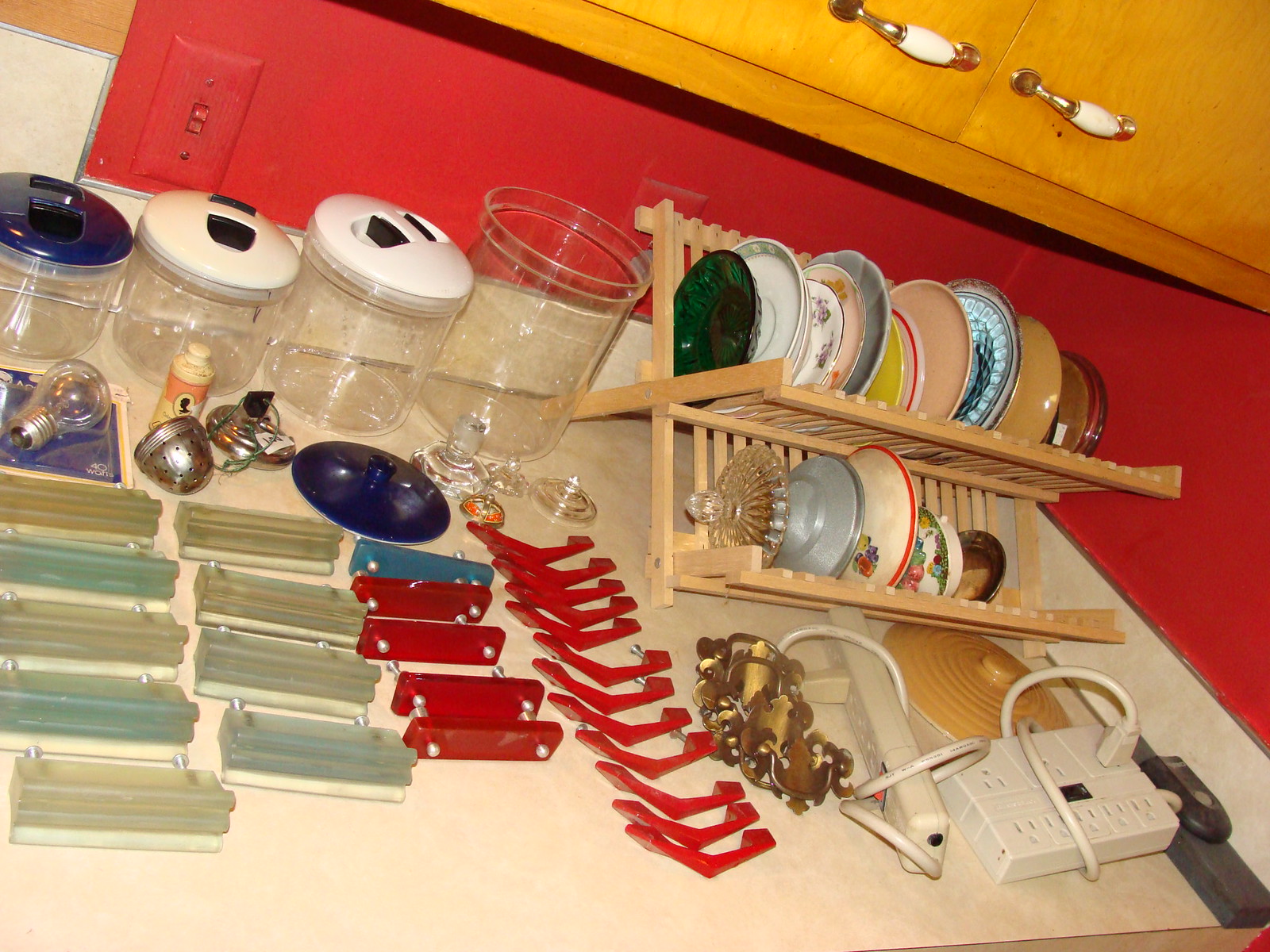In this vividly colored kitchen scene, the walls are painted a striking red, seamlessly extending to the light switch, which blends perfectly with the wall. Dominating the upper portion of the image are wooden cabinets, each fitted with two handles for easy access. These cabinets sit above a countertop cluttered with various items. A rack holds numerous plates and bowls; it is unclear whether this is their permanent storage place or simply where they are left to dry. Among these dishes, a recognizable candy dish top is also visible.

On the countertop below, several small plastic items are scattered, their exact purposes ambiguous. Further adding to the eclectic mix of objects are four empty canisters designed for storing powdered goods like sugar and flour. These canisters have a mix of covers—one blue, two in white and black, and the fourth cover seemingly misplaced on the counter. Additional details include a metal tea infuser, an unopened screw-in light bulb still in its packaging, and two power strips inexplicably plugged into themselves.

This kitchen snapshot captures a blend of vibrant color and everyday chaos, offering a glimpse into a busy and well-utilized space.